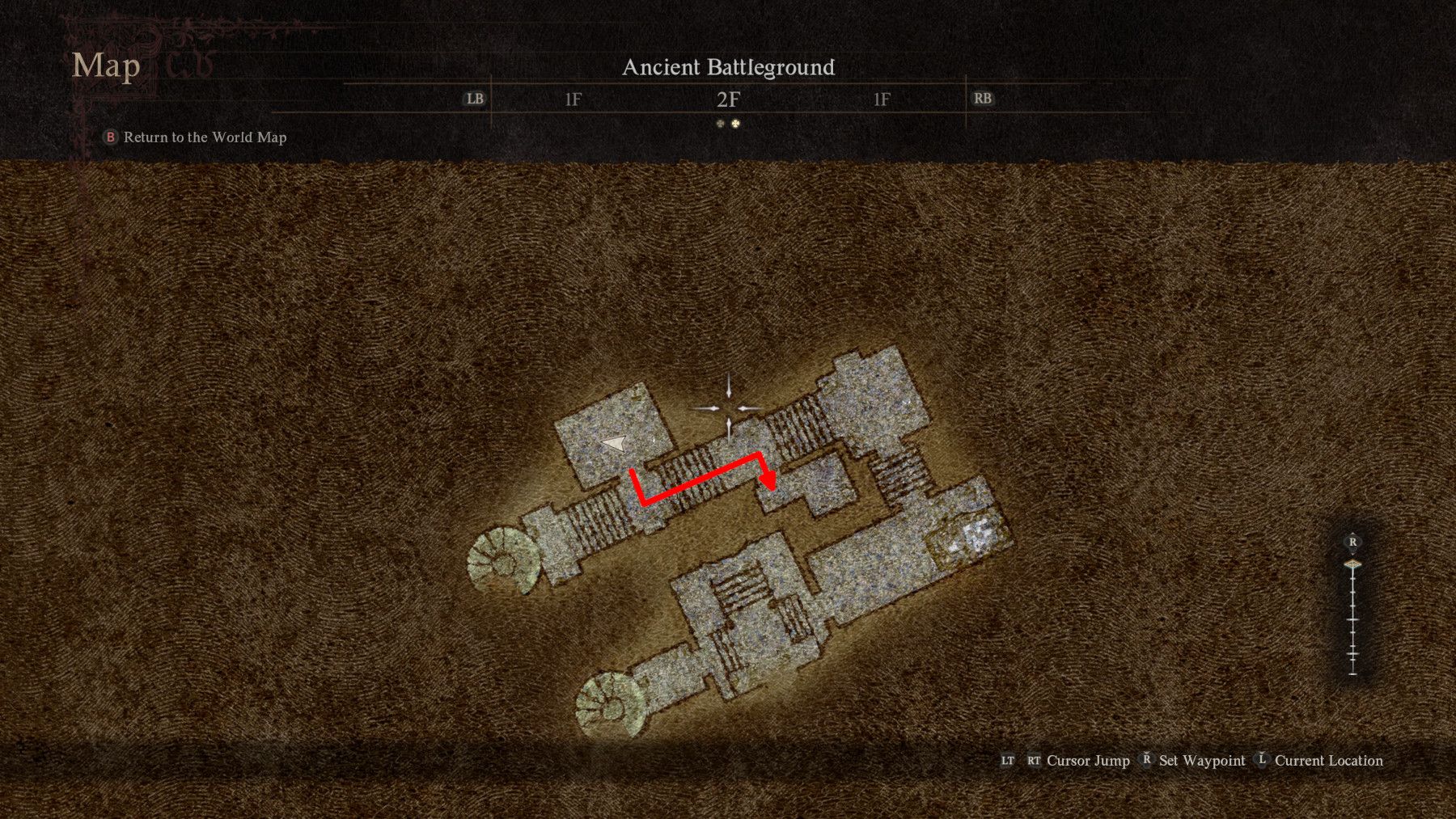This image is a detailed screenshot from a video game, depicting a complex floor plan overlaid on a brown, textured background that resembles fibrous carpet or dirt. The screen is bordered by a black frame with various UI elements. In the top right corner, grey text reads "Map", and underneath, there's a small red circle and the label "Ancient Battleground". Numbers such as "1F," "2F," and other identifiers are visible but somewhat blurred. 

The floor plan itself resembles a U-shaped structure, featuring a geometric layout akin to an architectural diagram. This layout includes multiple rooms and hallways, with a prominent red arrow navigating through the spaces. The ends of the U-shape house spiral or cylindrical staircases. On the left arm of the U, there is a series of rooms and a hallway, leading to a larger room at the central hinge. On the right arm, the stairs connect to a large rectangular room. Below this, another large common area, potentially an atrium, connects to additional rooms and another cylindrical structure.

Notable features include various circular elements on the outer edges, which appear to be staircases, and a white interior section indicative of an architectural diagram, possibly of a temple or house. The center of the screen features a cursor made of four white arrows forming a cross. At the bottom, there’s a faded black box with text in the right corner that reads "Cursor Jump," "Set Waypoint," and "Current Location," along with a slider likely used for game settings.